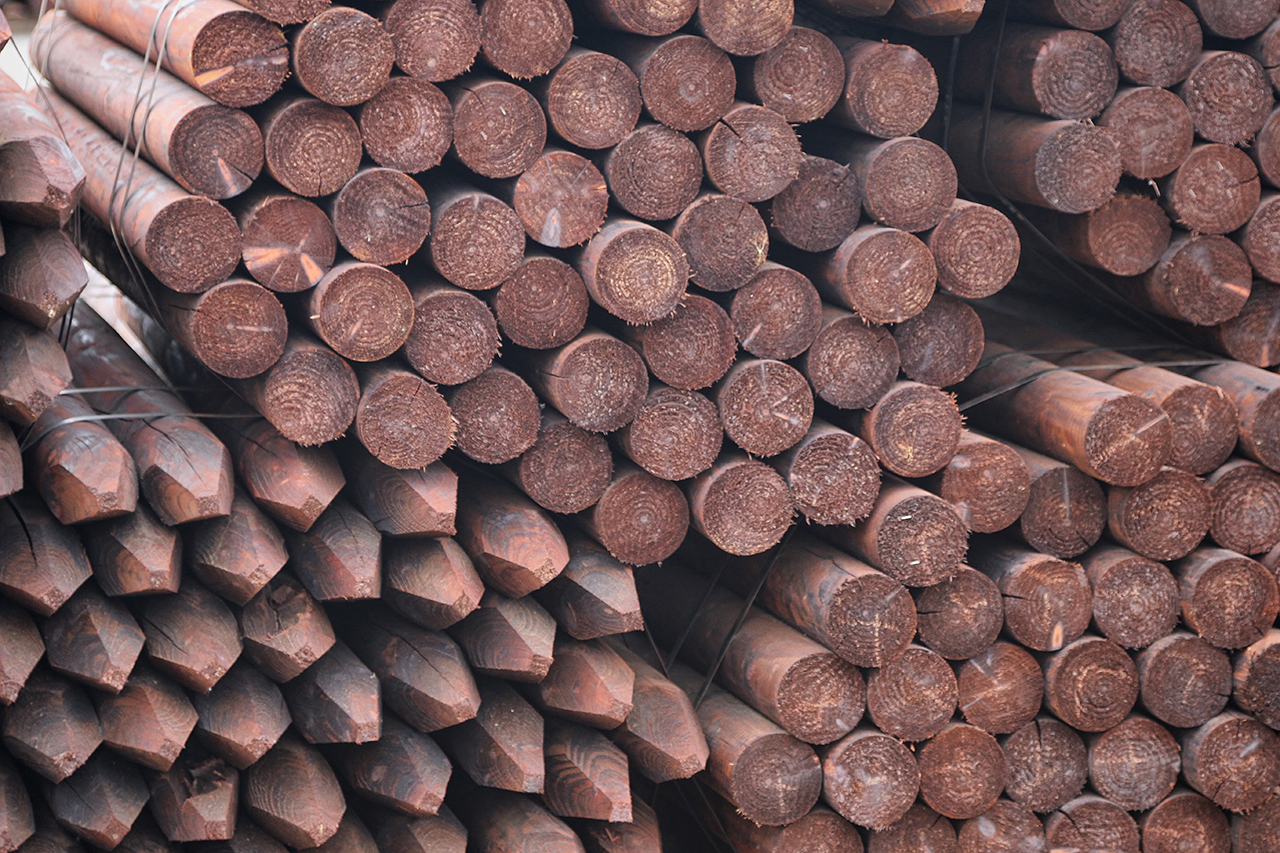This image depicts several bundles of large, cylindrical logs, likely processed for use as telephone poles. Arranged in four distinct piles, the ends of the logs are prominently displayed, revealing a mix of flat and pointed tips. The bundles are held together with dark black bindings. Due to the absence of a size reference, it's challenging to gauge their exact thickness, although they appear substantial. The logs, predominantly brown, have rough edges indicating recent milling. The lower-left bundle features logs with pointed ends, possibly intended for ground insertion, while the other bundles consist of logs with flat, round bases. The fourth bundle is partially visible in the upper right, with the other three more completely seen in the image's top left, bottom left, and bottom right corners.